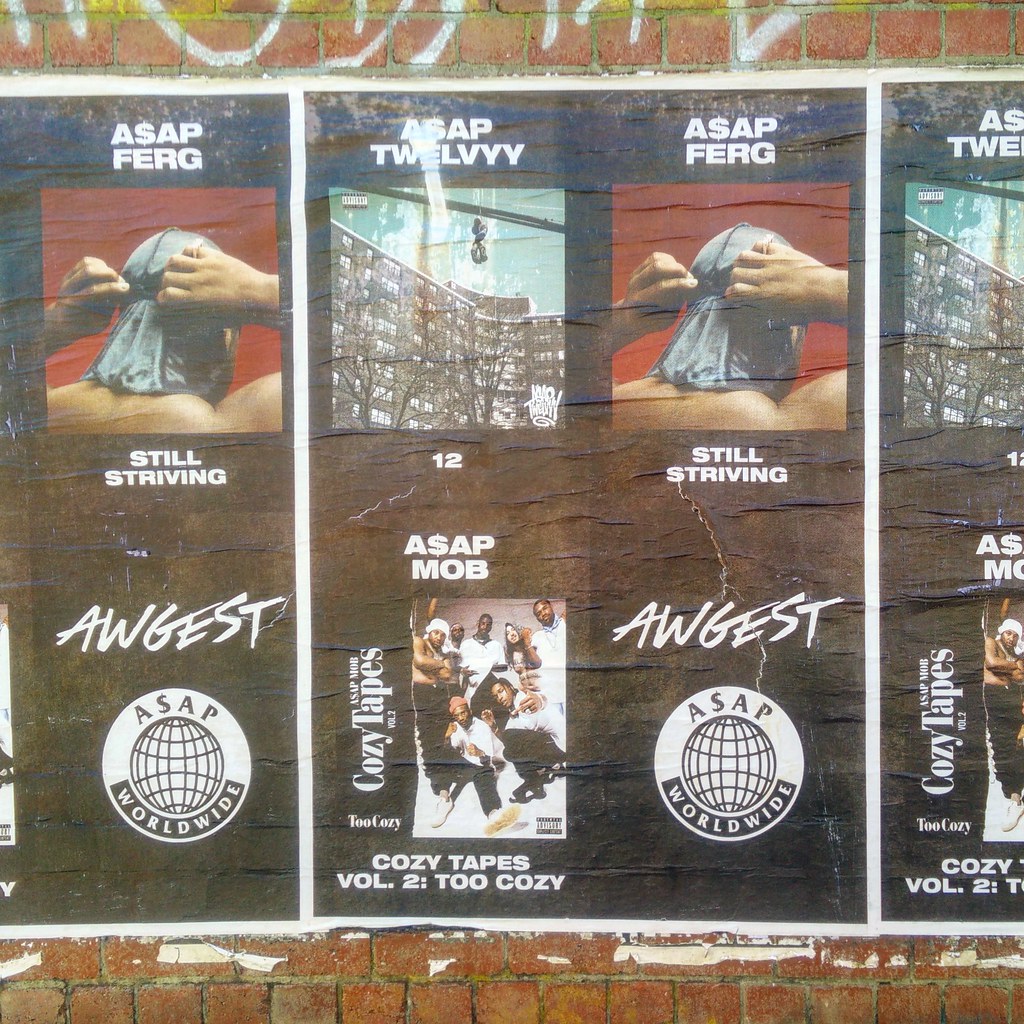The photograph captures an advertisement poster plastered on an old red brick wall with visible dirt in the grout and white graffiti in the upper left corner. The poster repeats in a series along the wall. Prominently, it promotes the music group ASAP Mob and its members, featuring the name ASAP Ferg with the phrase "Still Striving" and another mention of "August" and "ASAP Worldwide" with a logo of a globe and grid lines. At the top left, there's an image of a man adjusting a blue do-rag, obscuring his face. Below it, in the middle column, "ASAP 12E" is printed above an image of a tall apartment building. The bottom section displays "Cozy Tapes Volume 2: 2 Cozy" with a group of young black men, appearing to be rappers, standing together in focus. Overall, the poster conveys a vibrant urban and musical theme, emphasizing the affiliation with the globally recognized ASAP Mob collective.